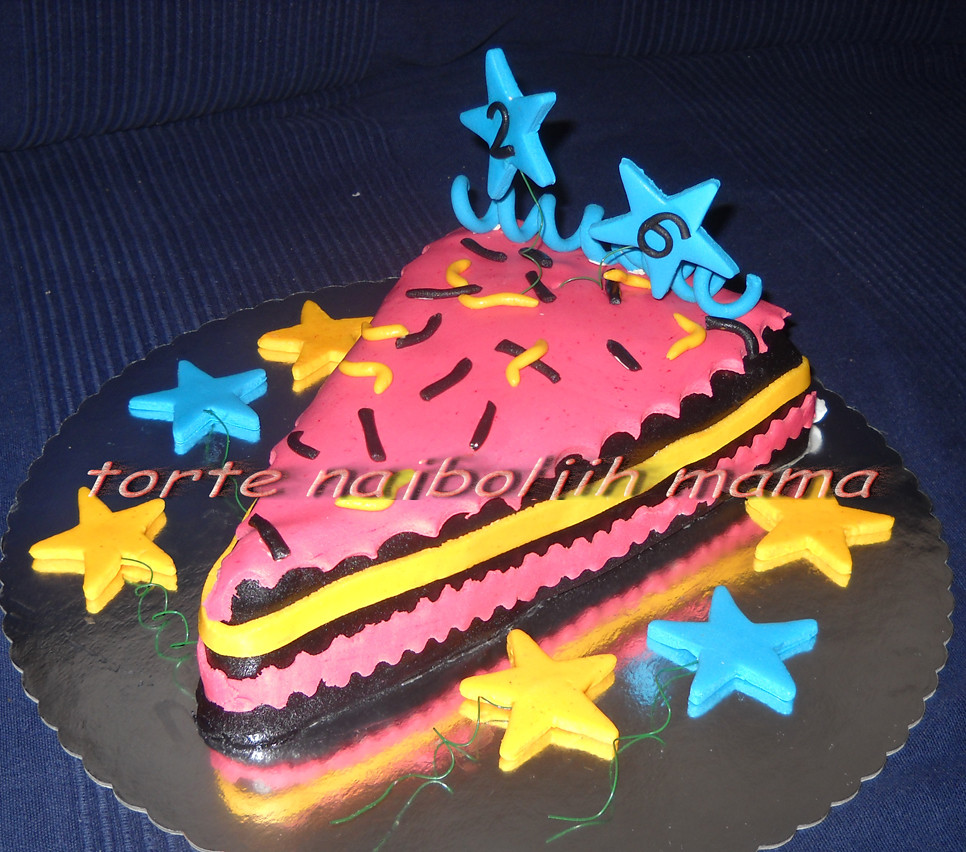This image features a close-up of a vibrant slice-shaped cake, prominently displayed on a silver cardboard platter, resembling those from a bakery. The cake, designed to mimic a cut slice, has a detailed, fondant-like icing that alternates between pink and yellow layers with hints of chocolate brown, creating a three-tiered pattern. The pink frosting on the top is adorned with large yellow and brown dots, mimicking sprinkles.

The cake rests on a table covered with a navy tablecloth, adding depth to the scene. Surrounding the cake are six alternating stars in yellow and blue, attached with wires and spaced evenly around the platter. The number "26" is displayed prominently on the cake with a "2" on one blue star and a "6" on another, suggesting a 26th birthday celebration. Additional details include a blue spiral embellishment at the back of the cake, enhancing its festive appearance.

Above the cake, text reading "Torte Nal Ibol Mama" is visible, possibly indicating a personal or cultural message related to the celebration. The cake's design, with its creatively cut edges and colorful decorations, aims to create an engaging and joyous birthday centerpiece.